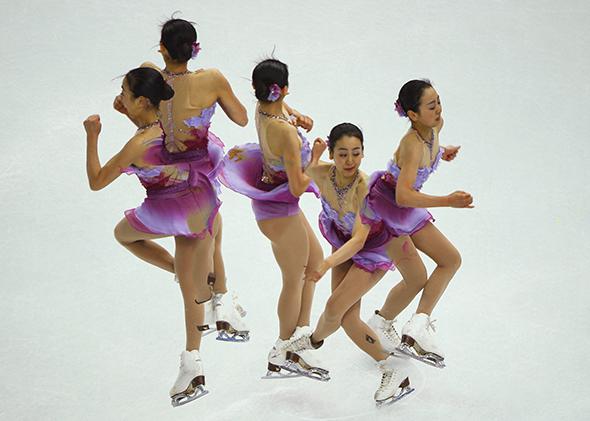The professionally-taken image on a white background captures five young Asian women, likely in their late teens, performing a synchronized ice-skating routine. Each skater is adorned in matching purple and pink costumes paired with white ice skates, complemented by dark hair neatly styled in buns with a purple flower accentuating their look. Their tan, flawless skin is further highlighted by identical jewelry - a purple and pink necklace around their necks. The skaters strike various dynamic positions, with some lifting and bending their knees, and others captured mid-twist, seemingly demonstrating the phases of a complex move. Despite the white ice being the only visible part of the rink, the coordinated elegance and mirrored appearances of the girls create an illusion of quintuplets or the same girl superimposed numerous times, underscoring the precision and harmony of their routine. There is no text in the image, enhancing the pure visual essence of their performance.